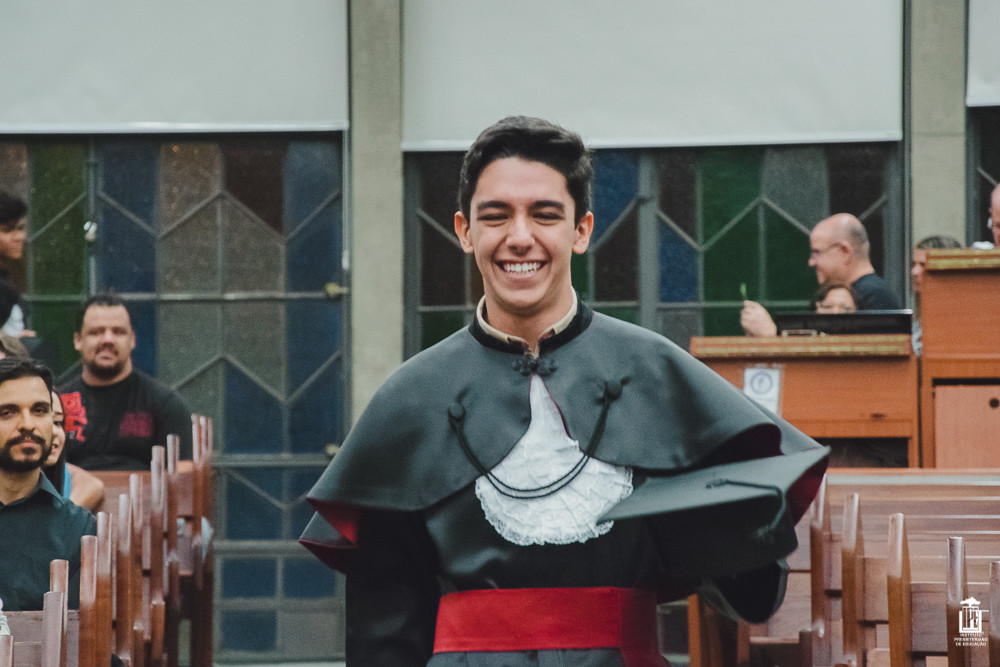This image captures a young man during a graduation ceremony, walking down the aisle of what appears to be a church, surrounded by wooden benches on both sides. He is positioned centrally in the frame, smiling directly at the camera. He is dressed in a black graduation cap, a black robe or cape over a white ruffled shirt, and a red sash. His dark hair is visible under the cap. Seated on the left side of the aisle are people, attentively looking towards the photographer. In the background, more families are gathered, some taking pictures. Two podiums are noticeable on the right side; one is manned by an older gentleman with glasses, possibly holding something, while the other, slightly higher, has two individuals partially visible behind it. The setting suggests an indoor space, likely a church, indicated by the presence of pews and stained glass windows. The scene is vibrant with various colors including white, gray, blue, dark red, purple, green, black, and brown.